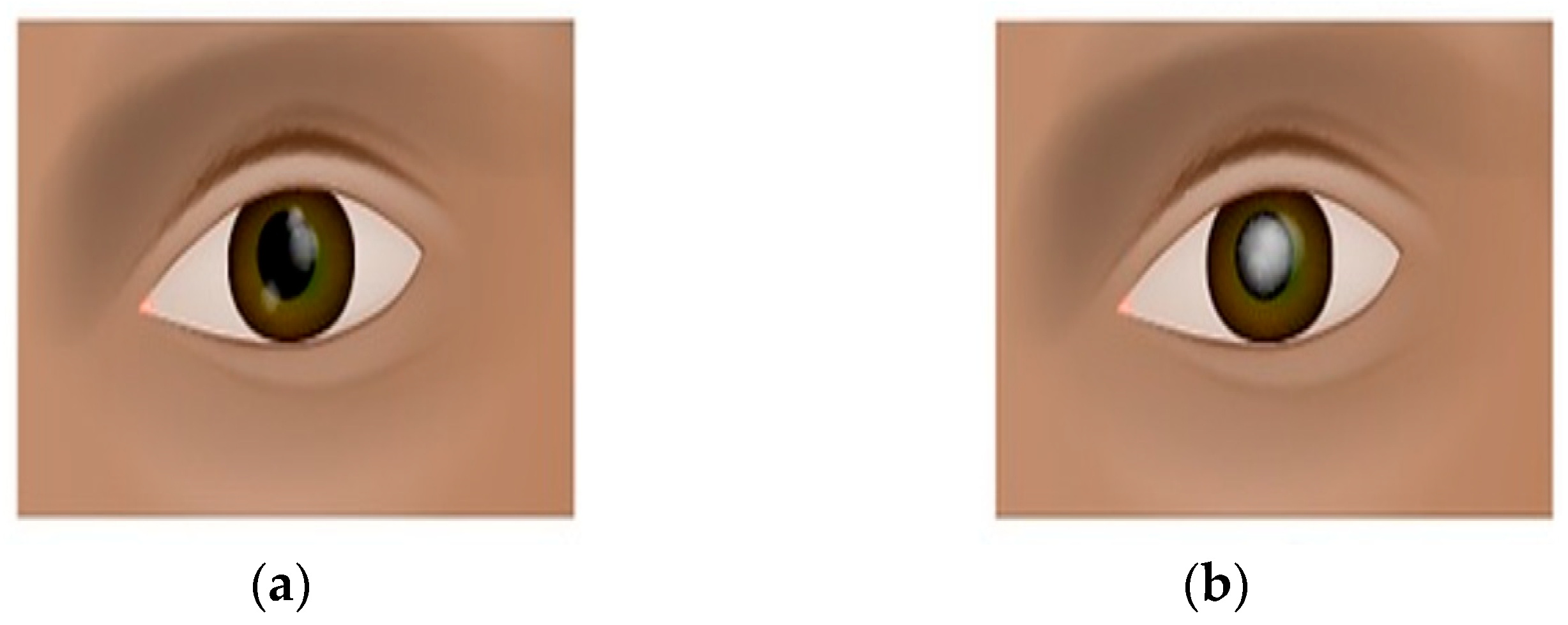This series consists of two detailed illustrations labeled "a" and "b" that depict human eyes against a light brown, golden skin tone background. Each image presents a close-up of an eye without eyelashes or eyebrows, emphasizing the eye itself. 

In illustration "a," the eye has a clear, dark brown iris with slight green tinging around the edges and a distinct black pupil, surrounded by the white sclera. In illustration "b," the same eye is represented, but the pupil appears white and cloudy, likely due to a condition such as cataracts. The iris remains light brown, similar to that in illustration "a." The images are drawn meticulously to highlight the differences in eye appearance, emphasizing the contrast between a healthy and a potentially diseased eye.